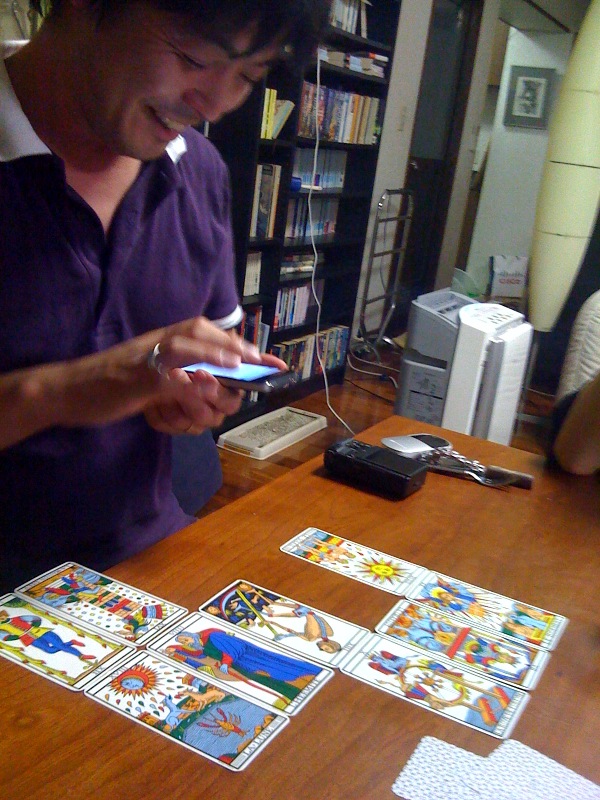In a cozy home office, an Asian man sits at a desk, fully absorbed in texting on his phone, a smile playing on his lips. His mouth is visible, showing his evident delight. The man is dressed in a purple short-sleeved shirt, and in front of him on the table lies an array of vibrant tarot cards, with their intricate designs turned up for display. Around nine of these cards, resplendent in hues of yellow, blue, and green, stand out vividly against the table's surface, while a few remain face down.

Sharing the table with him is another individual, a woman clad in a white blouse, her elbow resting casually on the table. Behind them, a bookshelf filled with DVDs and a tall white speaker or electronic device add to the room’s ambiance. The scene captures a moment of shared enjoyment and curiosity, as the man engrosses himself in his phone, exuding an air of happiness and contentment.